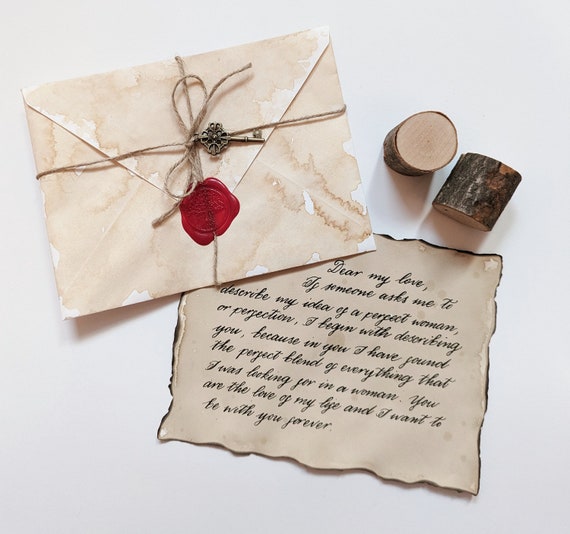A nostalgic and romantic scene unfolds in this photograph featuring an intimate love letter and its envelope, accompanied by two rustic corks. The corks exhibit a variegated appearance, with hues of blonde wood tinged with deep blacks and dark browns, resting elegantly on a pristine white surface. The letter, penned on ivory-colored paper that shows signs of age and wear, bears the marks of water damage with slight peeling and edges darkened to a blackish hue. Written in cursive with black ink, the heartfelt message begins with "Dear my love" and unfolds into a declaration of eternal affection and admiration.

Adding to the vintage charm, a distressed envelope lies atop a corner of the letter. The envelope is weathered with brown water stains and secured with both twine and a classic red wax seal. Atop the envelope rests a small, silver key, adding an element of mystery and timeless romance to the composition. Every detail of the photograph evokes a sense of age-old love and treasured memories, beautifully encapsulated in this tender arrangement.